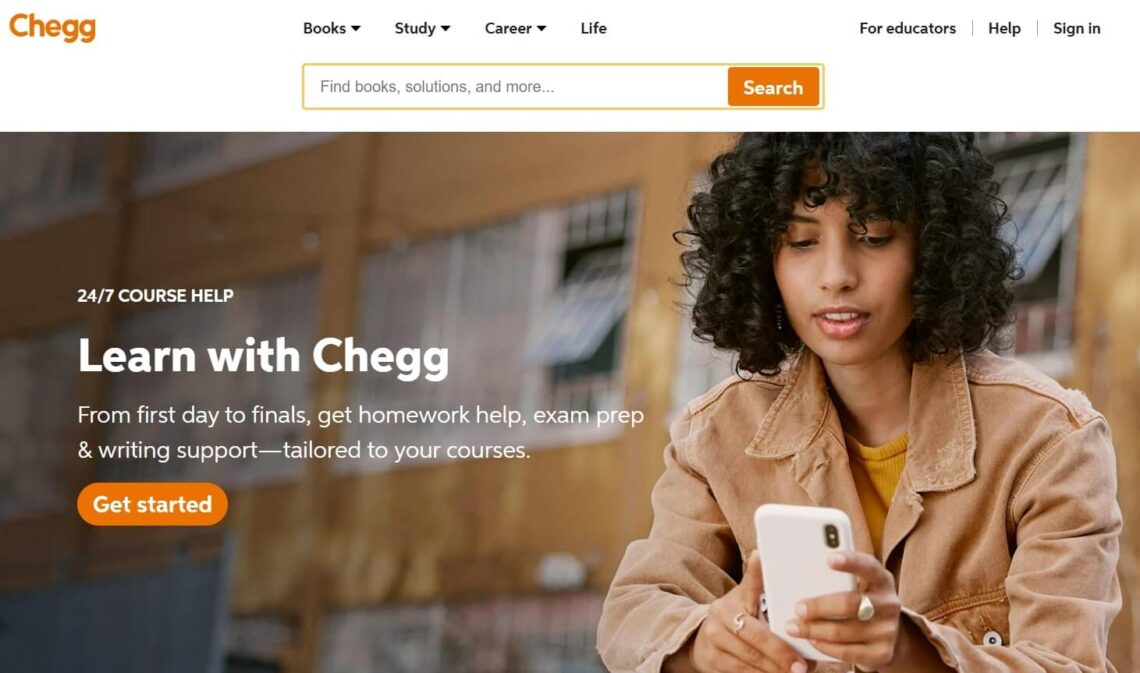This is a screenshot of the Chegg website. The top left corner features the Chegg logo prominently. In the central part of the top menu, there are several links titled "Books," "Study," "Careers," and "Life," each accompanied by a small downward-pointing triangle indicating a dropdown menu. Below this section, a search bar with the placeholder text "Find Books, Solutions, and More" is situated, with an orange button with white text adjacent to it. 

On the far right of the header menu bar, there are links for "For Educators," "Help," and "Sign In." 

Beneath the header is a large, eye-catching image of a young woman with dark, curly hair, possibly of Middle Eastern descent, in her early to mid-twenties. She is stylishly dressed in a tan denim jacket over a yellow sweater and is holding a cell phone, seemingly either taking a photo or browsing. 

To the side of the image, there is a textual call to action that reads, "24/7 Course Help. Learn with Chegg. From first day to finals, get homework help, exam prep, and writing support tailored to your courses." An orange "Get Started" button with white text is prominently displayed below.